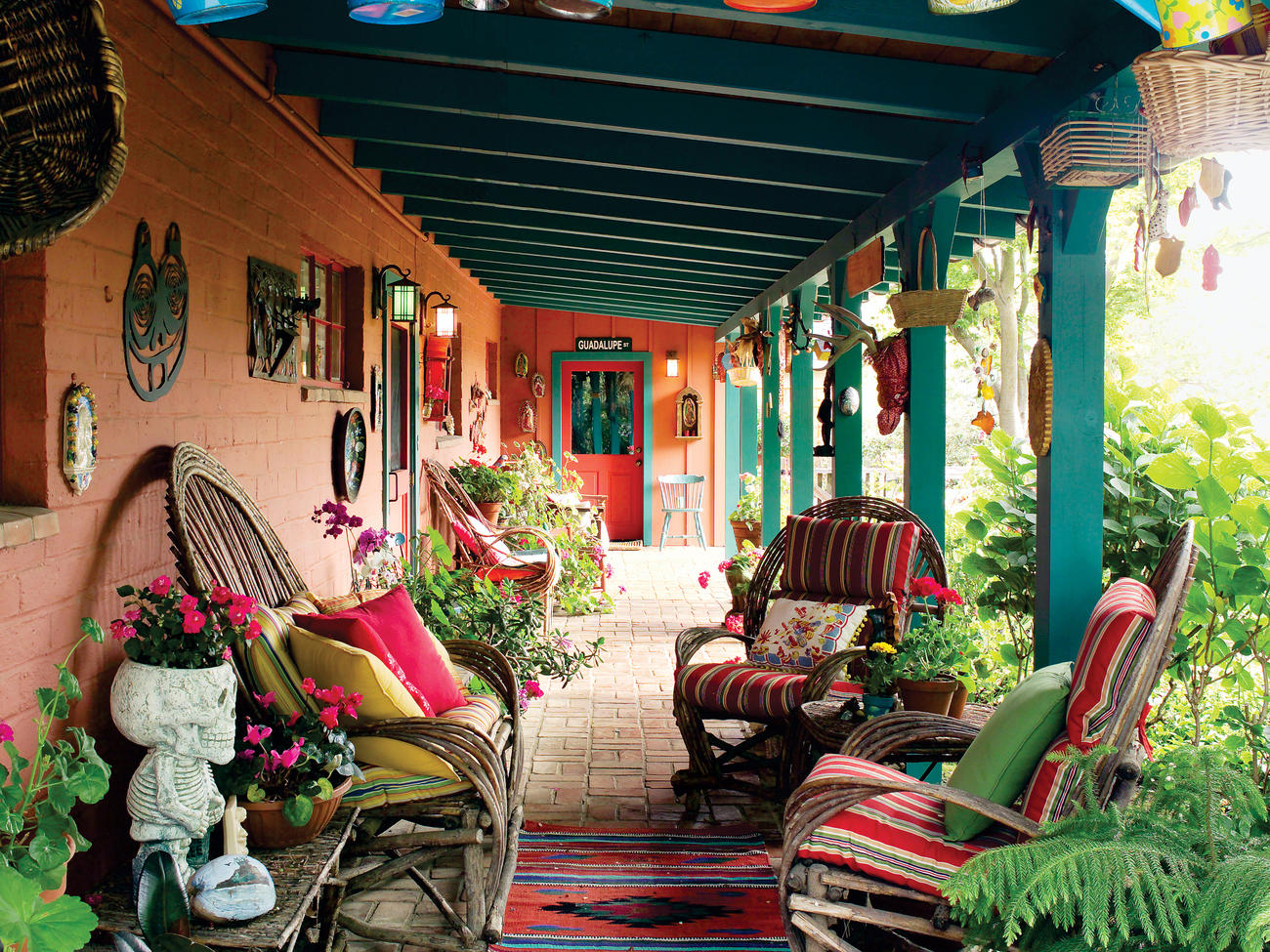This bright and colorful photograph captures a picturesque patio area with a vibrant Southwest feel, possibly located in a sunny region like Arizona, California, or Mexico. The patio, framed by pinkish-tan brick walls and a turquoise-painted wooden covering, features a rustic seating arrangement with three reclining chairs crafted from bent wooden sticks, each adorned with striped cushions. To the left of the image is an array of potted plants, including a distinctive Day of the Dead vase shaped like a skeleton's skull filled with flowers.

Above a red door on the left wall, a sign reads "Guadalupe Street," enhancing the authentic Southwestern ambiance. The space is further decorated with a Native American-style rug featuring red and blue patterns, several hanging baskets, and wind chimes, creating a cozy and culturally rich environment. Additional ornaments and foliage adorn both the wall and the surrounding area, completing the charming and eclectic aesthetic of this inviting patio.